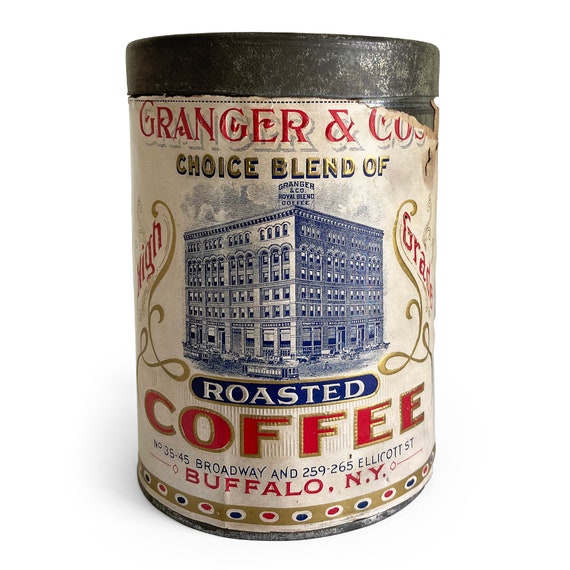This photograph features an antique tin of roasted coffee produced by Grainger & Co. The tin, which shows significant signs of age with a tarnished and weathered metal surface, remains intact despite the partial peeling of its paper label. The black-topped tin is adorned with a detailed label that reads: "Grainger and Co. Choice Blend of Roasted Coffee, 1935 to 45 Broadway, and 259 to 265 Ellicott Street, Buffalo, New York." An illustration of the Grainger and Co. Coffee Building is also depicted, showcasing a six-story structure with numerous windows. Notably, the fourth and fifth floors feature high, two-story tall arched windows, while the top floor has one-story tall arched windows arranged in groups of four. This historic tin, likely over a century old, reflects the rich legacy of Grainger & Co. and its Buffalo, New York origins.